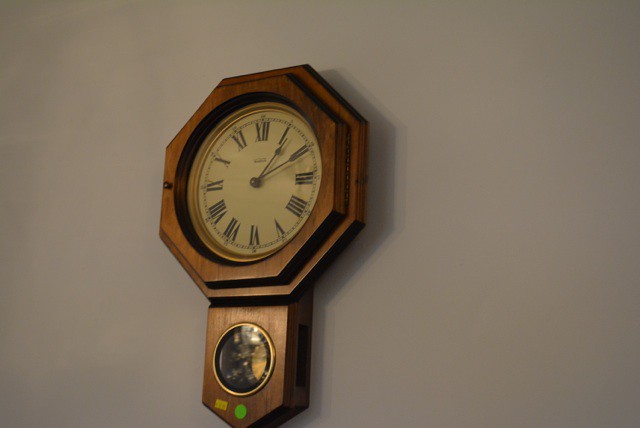This photograph showcases a wall-mounted clock designed with a medium brown wooden frame. The clock's frame is crafted into a hexagonal shape, adding a touch of geometric elegance to its rustic appearance. The primary clock face, which is round, is set within this hexagonal frame and features a creamy yellow background adorned with black Roman numerals and black clock hands, indicating the time as 1:10.

Extending from the bottom of the hexagonal frame is an additional wooden piece that supports a secondary round face. This secondary face is black and encircled by a thin gold band, though the details within the black face are indistinguishable due to the blurriness of the image. Directly beneath this black face, there is a green circular element, and adjacent to it is a triangular yellow price tag. The clock hangs against a stark white wall, further highlighting its detailed woodwork and intricate design.